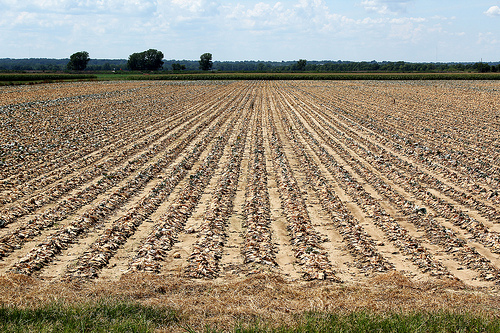In this detailed full-color photograph taken on a mostly sunny day with natural light, the viewer is presented with a freshly harvested farmer's field. The arid ground, a dry tan-brown color, stretches across the image, showcasing long, uniformly tilled rows where the bulk of the crops have been removed. In the foreground, a small patch of green grass is intermixed with various yellow, dried grasses, highlighting the transition from cultivated land to uncultivated areas. Off in the distance, a square hedgerow frames the field, delineating it from other sections.

Beyond the hedgerow lies a flat green expanse dotted with multiple trees, leading to a more distant tree line that separates the land from the horizon. Above, the light blue sky is punctuated by scattered white clouds, adding depth and contrast to the otherwise earthy tones of the landscape below. The photograph captures the aftermath of the harvest, with the barren yet meticulously aligned rows of the field reflecting both agricultural precision and the passage of the growing season.